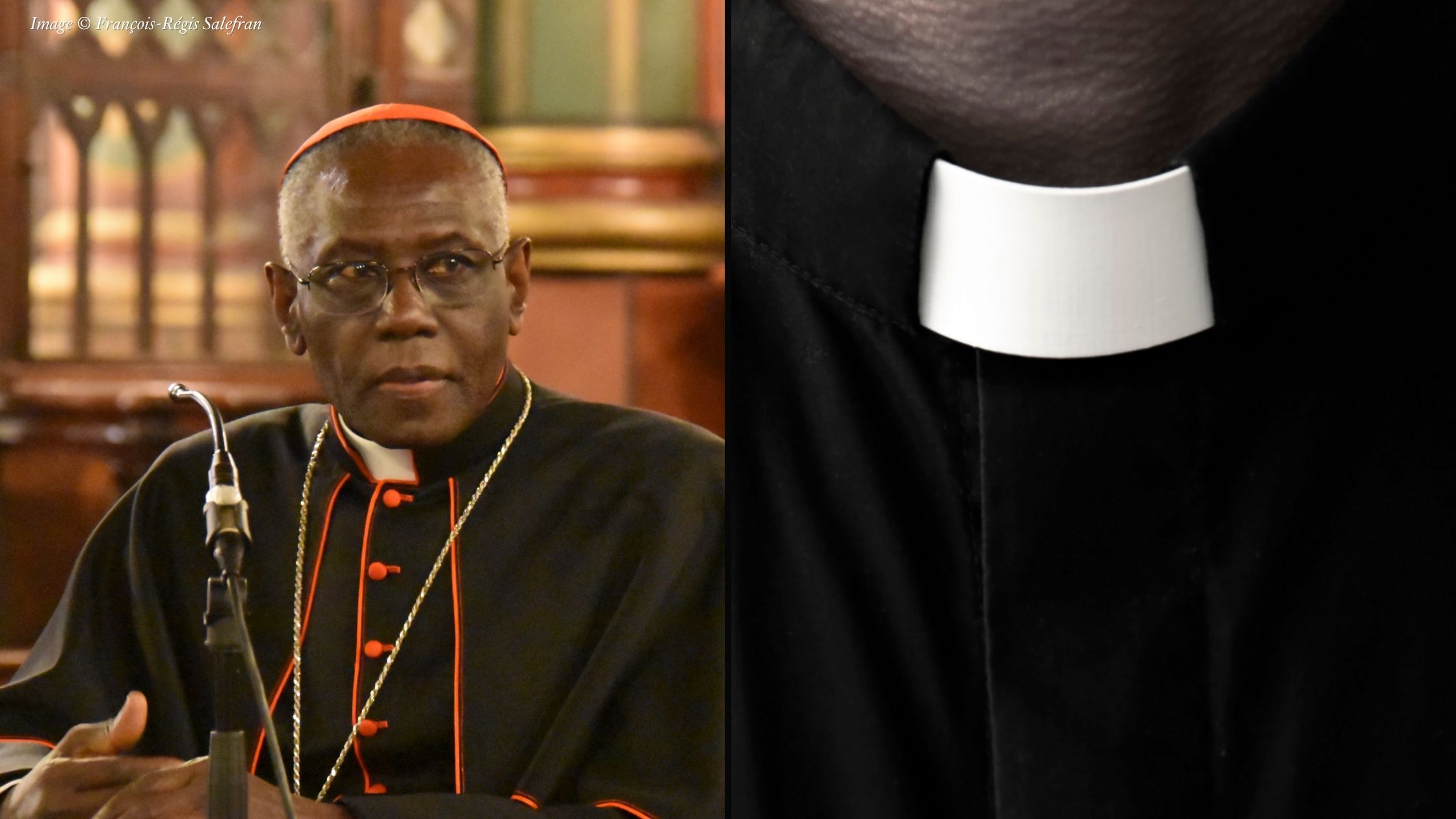The composite photograph depicts two distinct images side by side, each showcasing aspects of Catholic priesthood. On the left, an African-American cardinal is seated, dressed in full cardinal regalia that includes a red-trimmed robe and a red zucchetto (beanie). He is wearing glasses and appears to be ready to address a congregation, positioned behind a microphone with his hands resting on an unseen table, and a blurred stained glass window in the background indicating a church setting. The right side features a close-up of a clerical collar on a black shirt, capturing only the collar and a small portion of the neck. Accompanying the images is a small text at the top left corner, credited to François-Régis Saffron, likely in French. The juxtaposition of the cardinal's poised figure and the symbolic collar emphasizes the solemnity and dignity of his clerical role.